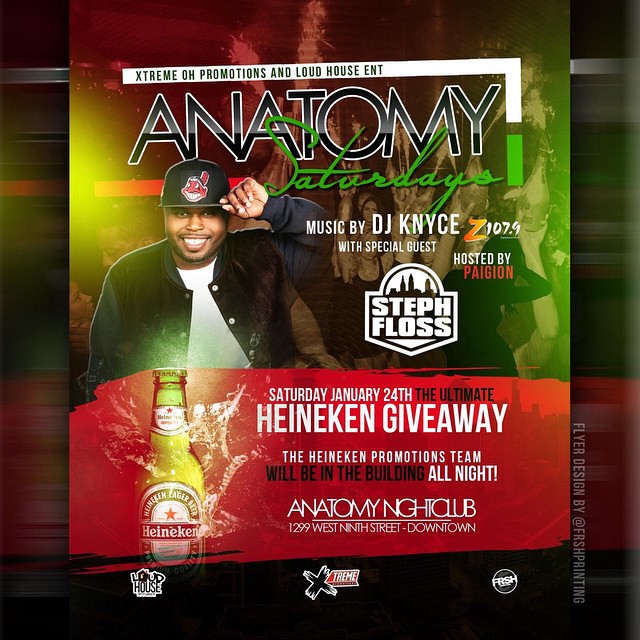This is a detailed photograph of a promotional flyer for "Anatomy Saturdays," featuring a vibrant background of dancing people with lit bottles of champagne and sparklers. The top of the flyer showcases a white rectangular border forming an L shape, prominently bearing the logos of "Extreme O Promotions" and "Loud House Entertainment." Centered within this border, the text "Anatomy" is displayed in bold black lettering with a white outline, while "Saturdays" is elegantly scripted in green cursive.

To the right, a young African-American man is depicted wearing a white shirt under a black jacket, while his left hand touches the brim of a black Cleveland Indians cap. Beneath this image, it reads "Music by DJ KNYCE" in bold font, accompanied by "Special Guest Steph Floss." The text "Z 107.9" appears nearby, indicating that the event is hosted by PAIGION and Steph Floss, whose logo is also featured.

Towards the lower part of the flyer, a red background frames a vibrant Heineken bottle splashing out of water, advertising the "Ultimate Heineken Giveaway" that will occur on Saturday, January 24th. The caption emphasizes that the Heineken Promotions team will be present all night at the event held at Anatomy Nightclub, located at 1299 West 9th Street, downtown. The bottom section of the flyer includes three logos: Loud House on the left, Extreme in the center, and FRSH on the right, alongside a side note stating "Flyer Design by FRSH Printing."